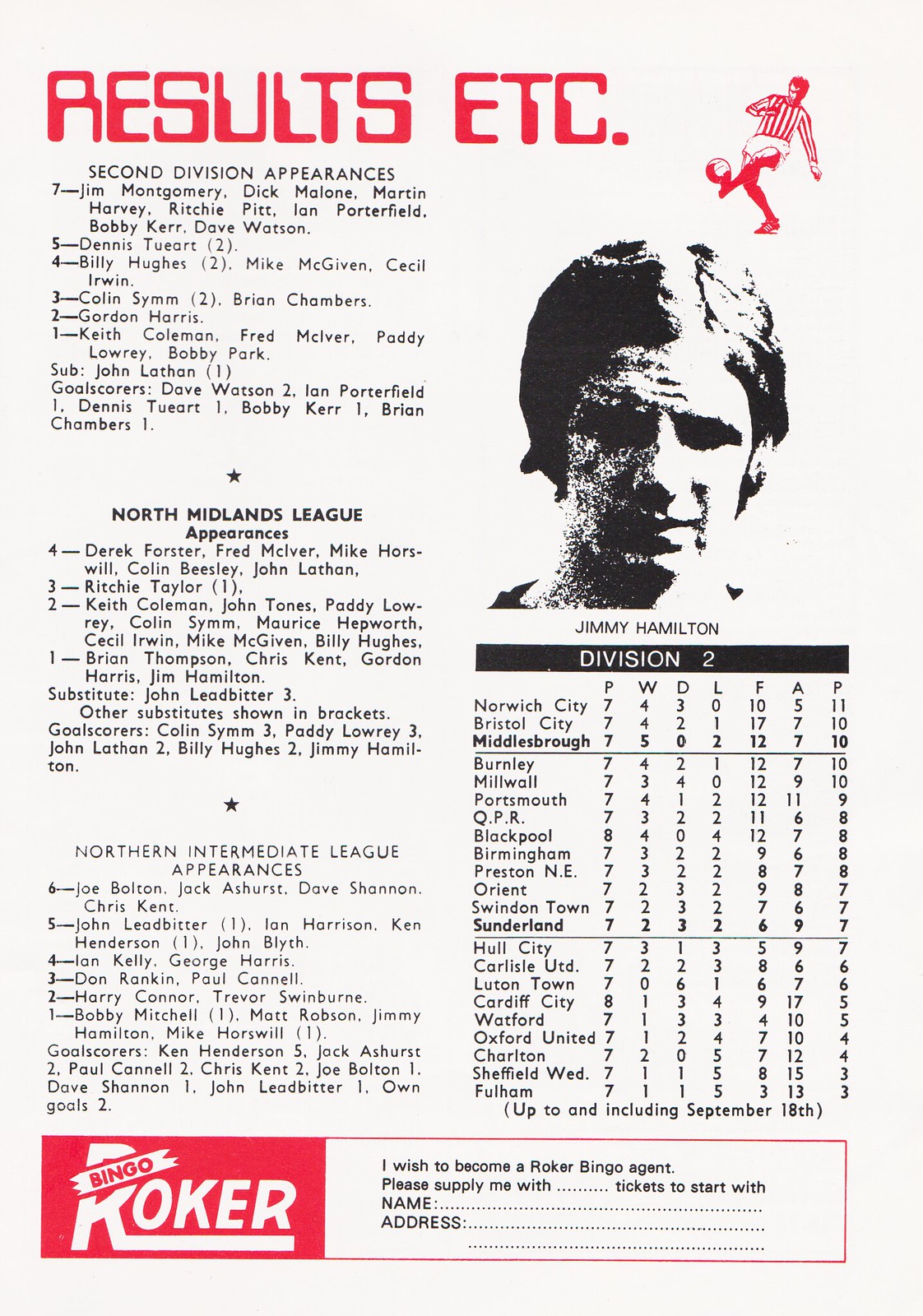The image depicts a detailed page from a football program with sections dedicated to player statistics and promotional content. At the top, bold red letters announce "Results, etc." in an old 80s computer-style font, accompanied by a red logo depicting a football player kicking a ball. Below this header, the page is divided into several sections: the first lists "Second Division Appearances" followed by individual player names, the second outlines "North Midlands League Appearances" with another list of players, and the third lists "Northern Intermediate League Appearances" with further player names. To the right, a black and white photo of a football player named Jimmy Hamilton is prominently displayed above the standings for Division 2, enumerating various teams and their current statistics. At the bottom of the page, a red rectangle houses an advertisement for "Roker Bingo," which includes a form stating, "I wish to become a Roker Bingo agent. Please supply me with ... tickets to start with," alongside fields for the reader to enter their name and address.